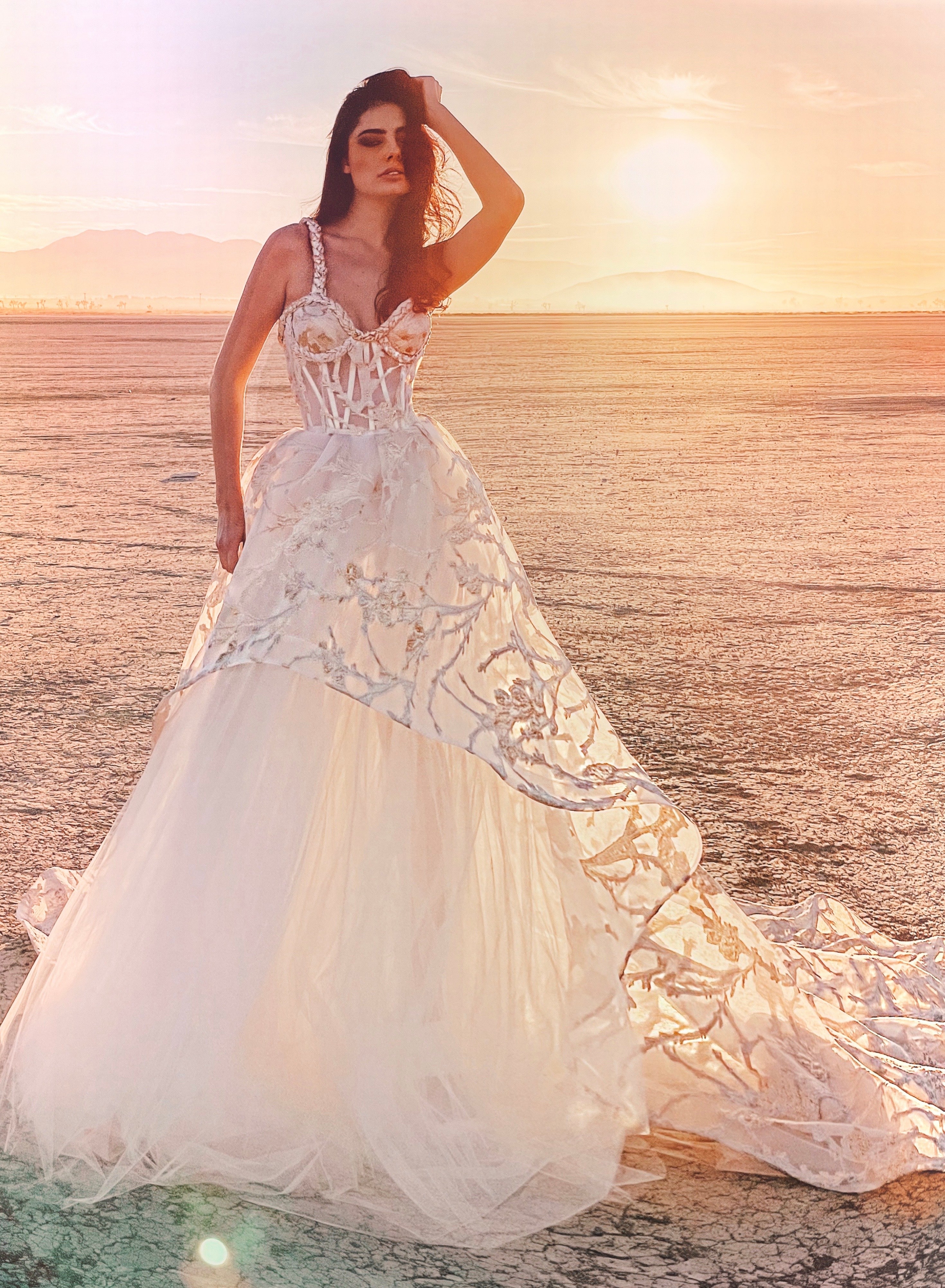A stunning portrait photograph captures a beautiful young woman in her early 20s standing upright in an expansive desert or salt flat, bathed in the warm, orangish glow of either sunrise or sunset. She strikes an elegant pose, with her left arm raised to touch her forehead and her right arm extended downward. The backdrop features distant hazy mountains and bright sunlight shining toward the viewer. The woman's wedding dress is a masterpiece of high fashion, featuring thin straps over her shoulders and a boned corset adorned with flower print lace. The brassiere part of the dress boasts woven, braided fabric around the cups, creating a unique and classy appearance. The dress, though form-fitting at the top, transforms into a voluminous skirt of delicate tulle with a high-low hem embellished with intricate lace designs. Unusually, the train extends mostly to her left side, lending an artistic flair to the garment. The sunlight filters through the porous fabric of the dress, highlighting its ornate details and adding to the ethereal quality of the scene.